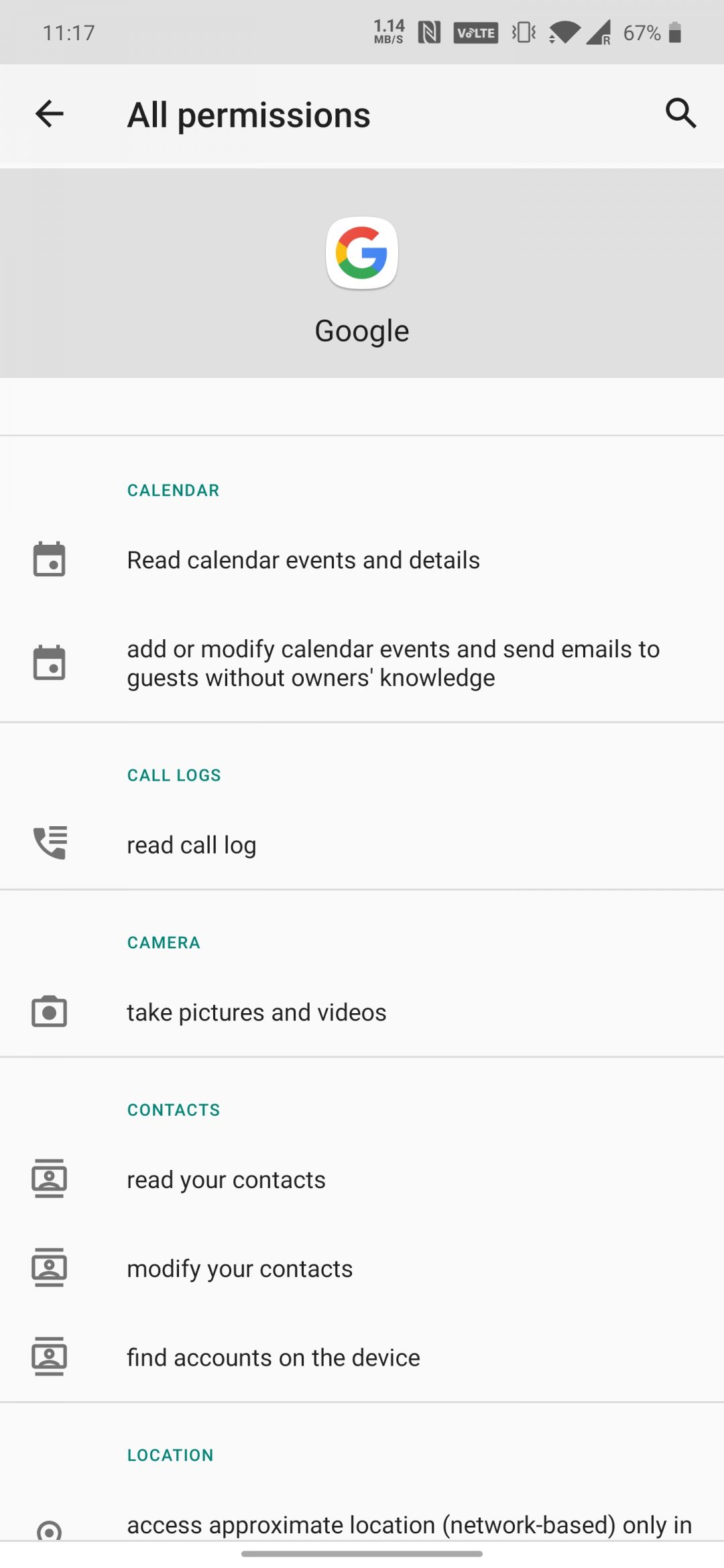This image is a screenshot displaying the permissions page of an application. At the top, there is a navigation bar with a back arrow labeled "All Permissions" and a search icon on the right side. The center of the screen prominently features the Google logo. Below the logo, the permissions are categorized into several sections:

1. **Calendar**: 
   - Read calendar events and details
   - Add or modify calendar events, and send emails to guests without the owner's knowledge

2. **Call Logs**:
   - Read call log

3. **Camera**:
   - Take pictures and videos

4. **Contacts**:
   - Read your contacts
   - Modify your contacts
   - Find accounts on the device

5. **Location**:
   - Access approximate location (network-based only), though the rest of the location-related text is truncated.

At the very top of the screenshot, the device's status bar shows the time as 11:17, the battery level at 67%, and a full WiFi signal.